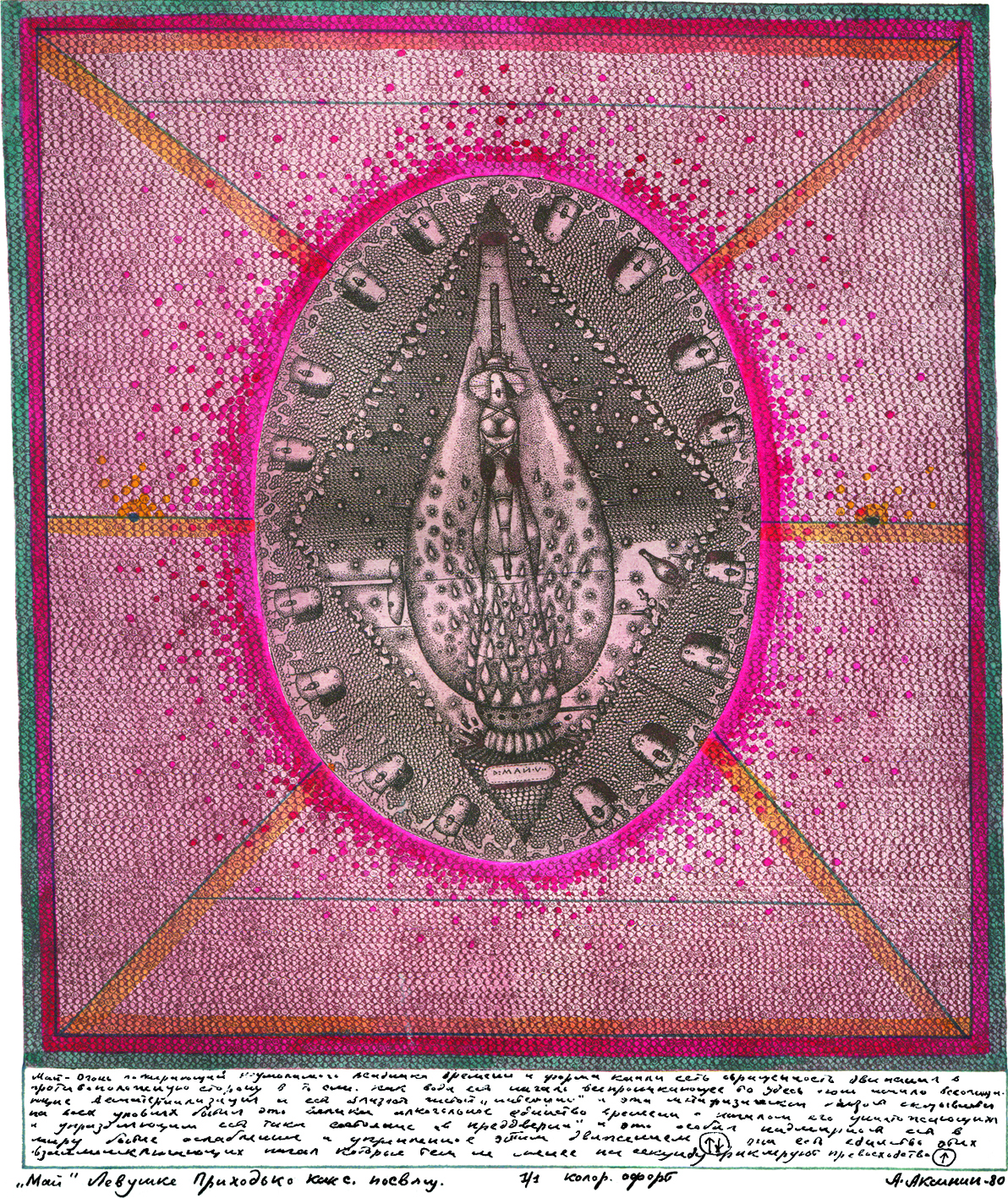The image is a highly detailed and unique piece of artwork that resembles an intricate piece of embroidery or a wall hanging. At the very center of the work is an abstract, almost pear-shaped, or lamp-shaped creature that is elongated, not quite humanoid, with a face and possibly a hat on top. Surrounding this central figure are numerous tiny flames directed outward. This central scene is encapsulated within a diamond shape, adorned with floating dots and various small objects. Encircling this diamond is an oval filled with faces similar to the central creature's.

This entire composition is then contained within a larger rectangle, featuring orange and yellow lines interspersed with pink hues. The outermost border of the image is a smaller green rectangle, framing the entire scene. The intricate, detailed central elements are rendered in grayscale, giving a sketched appearance, while the broader surrounding areas exhibit vibrant colors such as teal, red, orange, and pink.

The artwork's base contains writing, which is too small to discern clearly. The overall impression is that of a beaded, textured piece, possibly grainy in resolution, yet striking for its bizarre, multidimensional craftsmanship.